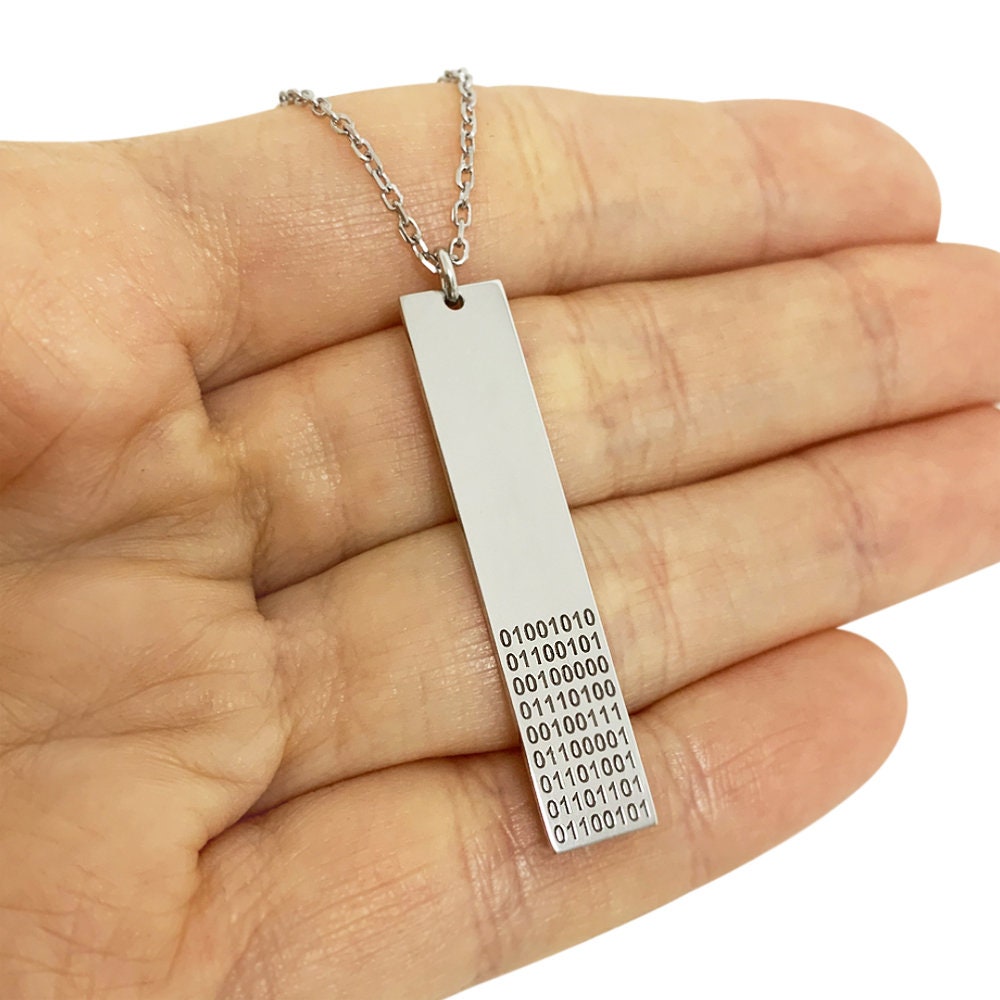The photograph captures a detailed close-up of a Caucasian person's left hand with the thumb out of the frame. The four visible fingers—index, middle, ring, and pinky—are tightly held together in a position as if about to shake hands. Draped around the index finger is a delicate silver chain link necklace adorned with a distinctive rectangular charm. This long, metallic charm extends from the middle finger down halfway to the pinky. The top half of the charm is plain, while the bottom half is intricately inscribed with rows of binary numbers: "01001010" and continuing with nine rows of intricate 0s and 1s, forming a unique pattern that suggests a computer code. The background of the photograph is entirely white, emphasizing the hand and the detailed binary-etched charm.